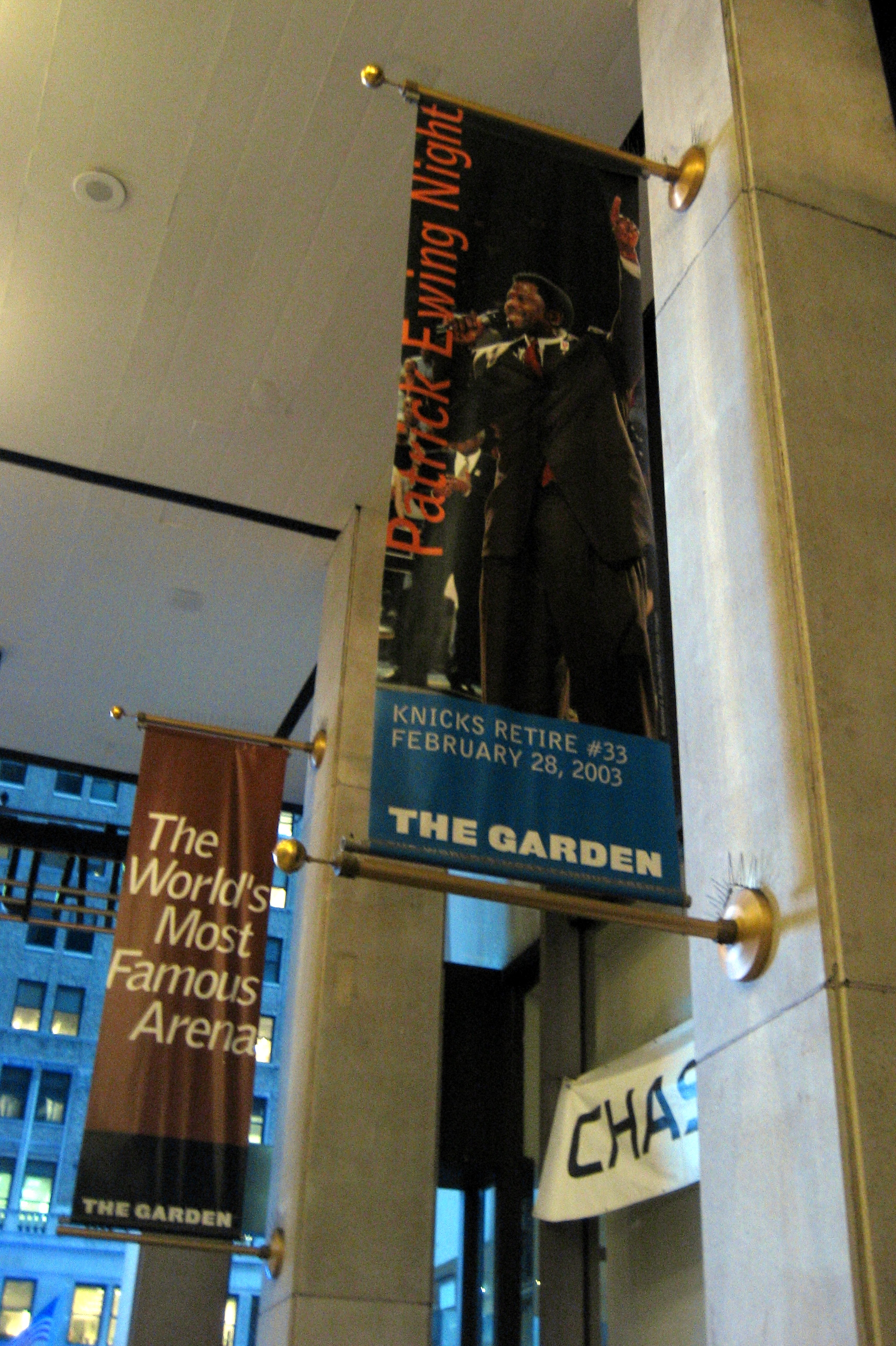This vertical rectangular image depicts the interior of Madison Square Garden in New York City. The photograph captures tall stone walls and windows, with various banners and advertisements adorning the space. A large white cloth banner prominently displays "C-H-A-S," indicating the presence of Chase Bank, known to have a branch inside Madison Square Garden. Flanking this banner are two gold posts supporting flags. The left flag reads "The World's Most Famous Arena, The Garden," while the right flag showcases a photograph of Patrick Ewing, labeled "Knicks Retire Number 33, February 28, 2003, The Garden." This nod to New York Knicks history highlights Ewing's celebrated career. A glimpse out the window reveals a towering skyscraper, further confirming the iconic New York City setting.